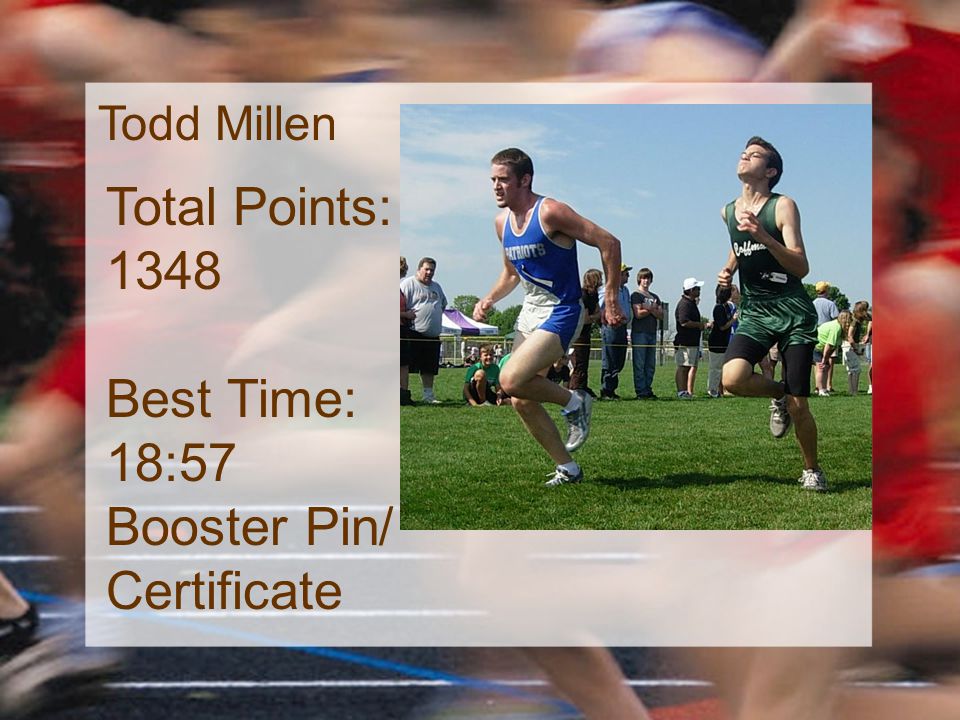The image depicts a lively outdoor cross-country race, featuring two prominent runners in the foreground. The runner on the left is clad in a blue and white uniform, paired with white and silver shoes, while the runner on the right sports a green and white outfit with black spandex. Behind them, a blurred crowd of spectators lines the sidelines of the grassy track, separated by a yellow rope. The background is adorned with a bright blue sky and a purple and white tent towards the left. In the upper left corner of the image, text reads, "Todd Millen, Total Points: 1,348, Best Time: 18:57, Booster Pin, Certificate." The scene captures the essence of a competitive race on a sunny day, punctuated by colorful attire and enthusiastic onlookers. The entire image is square, with a smaller, also square, inset photograph slightly off-center to the right, and text positioned on the left side.